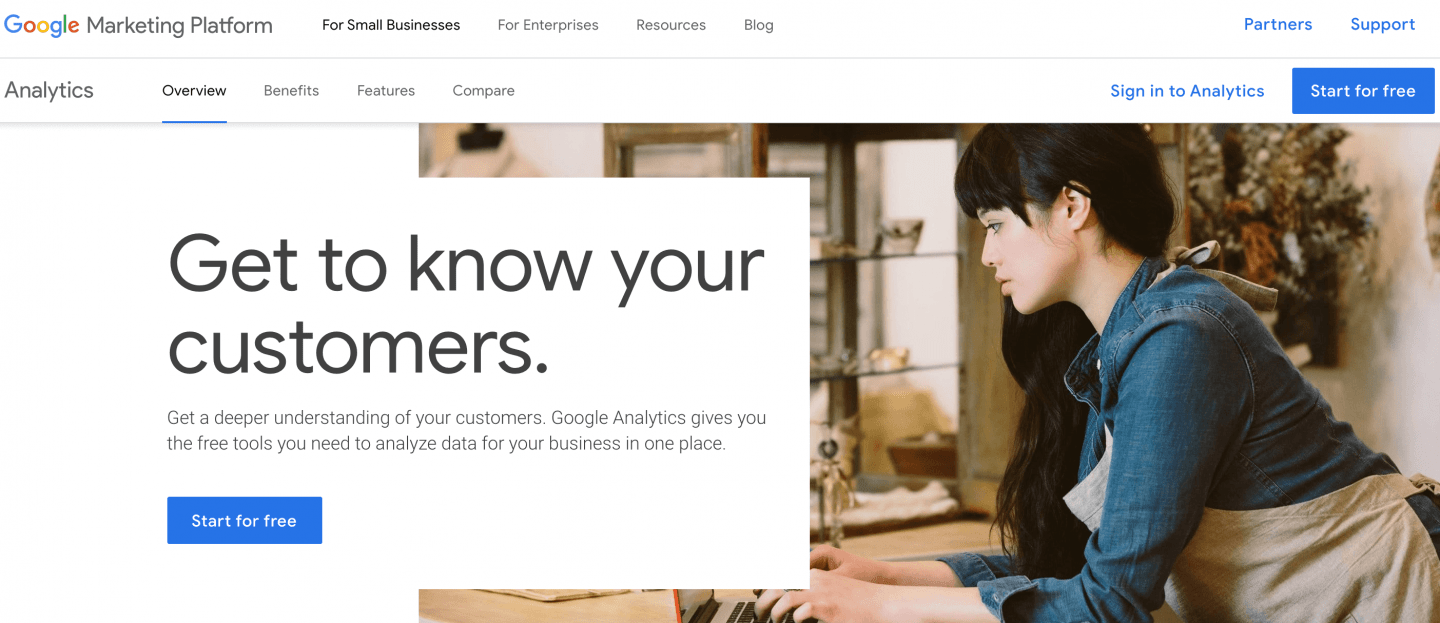A woman wearing a blue jean jacket and a brown apron is focused on typing on her laptop against a clean, white background. The laptop screen displays a message promoting Google Analytics: "Get to know your customers. Get a deeper understanding of your customers. Google Analytics gives you the free tools you need to analyze data for your business in one place." Above the message, the Google Marketing Platform banner is visible, featuring options such as "For Small Businesses," "For Enterprises," "Resources," "Blog," "Partners," and "Support," all highlighted in blue. The "Analytics Overview" section is underlined, indicating it is selected. Additional options like "Benefits," "Features," and "Sign In to Analytics" are also in blue. A prominent blue rectangle button at the bottom of the screen reads "Start for free" in white text.